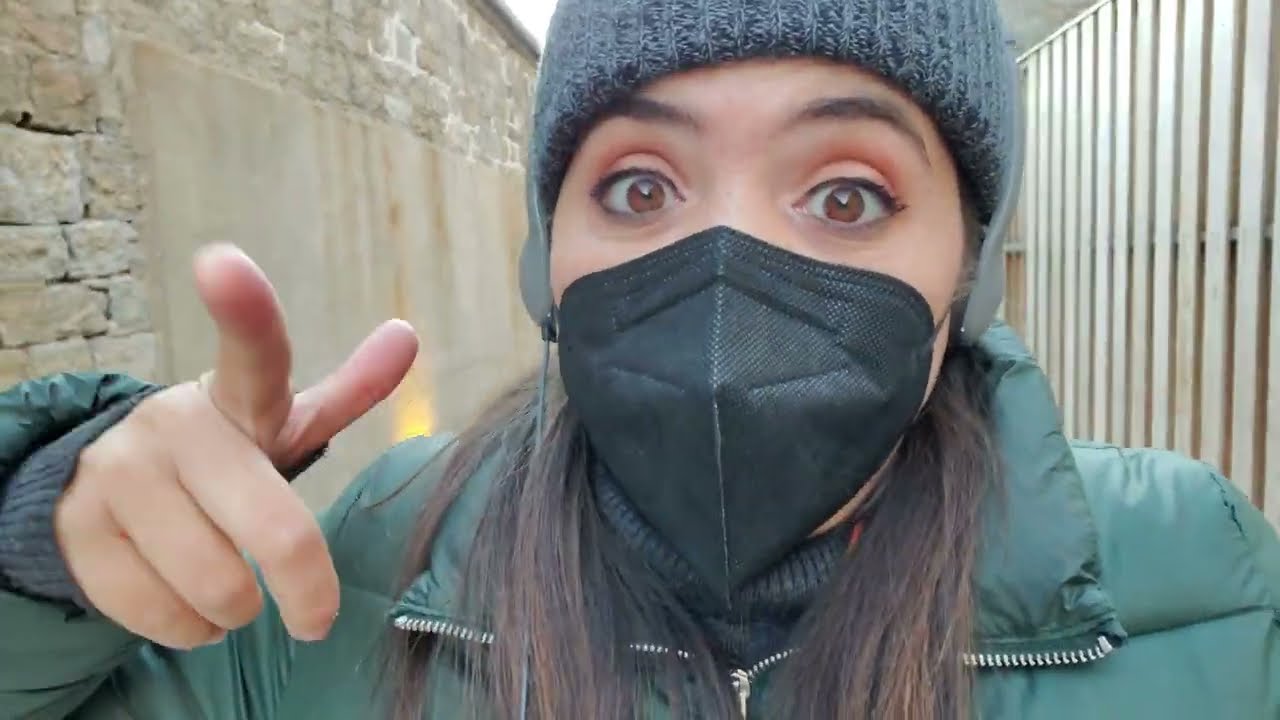In this horizontal, rectangular image, a woman stands in front of a contrasting backdrop featuring a beige brick wall on her left and vertical metal panels on her right. The woman, possibly white or Middle Eastern, has her brown hair partly concealed by a dark blue beanie. She wears a black medical mask and a green puffy winter jacket over a greenish turtleneck. Her wide, expressive brown eyes are directed at the camera. Her right hand, positioned on the left side of the image, points towards the viewer with her index finger. She appears to be wearing headphones under her beanie, and her surprised expression hints at the circumstances surrounding the photo.